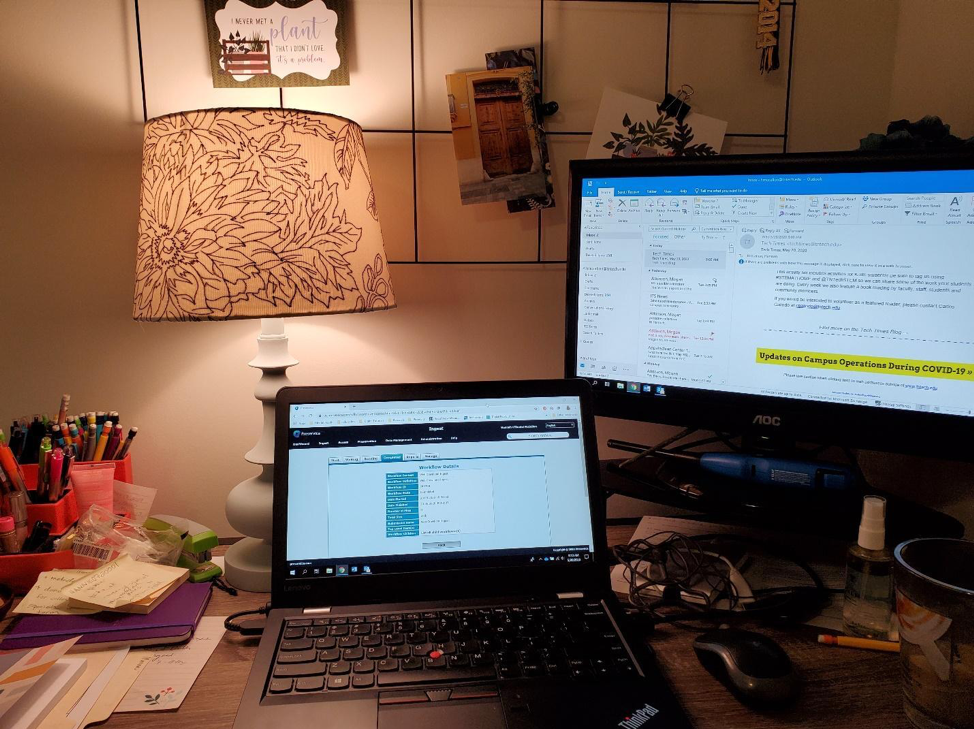The image depicts a cluttered desk situated in the corner of a room, likely viewed from the vantage point of a chair. On the left side, there are two small caddies, one red and the other pink, brimming with mechanical pencils, pens, and possibly highlighters. Adjacent to these, several plastic bags contain miscellaneous items, contributing to a somewhat disorganized appearance. 

A purple notebook and sticky notes with handwritten annotations are scattered across the desk, alongside a file folder and other assorted objects. A laptop, identified as a ThinkPad, is positioned in the center and is connected to a power source. Directly behind the laptop, an illuminated desk lamp provides the primary light source, given that the overhead light is not turned on.

In the background, a bulletin board adorned with various items, including magnetic cards, is mounted on the wall. To the right of the laptop, a significantly larger monitor displays a screen with the text "Campus Operations During COVID-19." A mouse is also present beside this larger screen. The overall setup appears to be somewhat messy, emphasizing the busy, lived-in nature of the workspace.